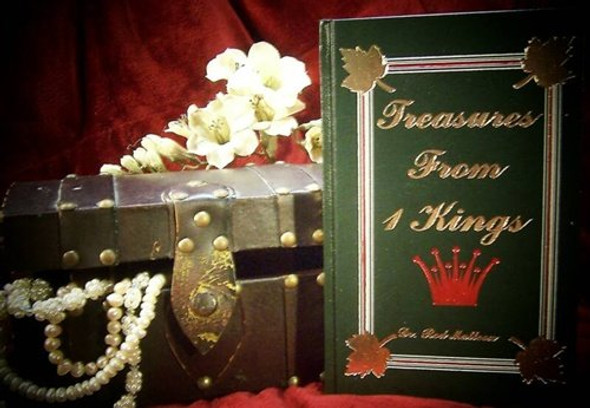The image features an intricately detailed scene set against a rich red velvet fabric backdrop. On the left side of the image, a partially open, black leather treasure chest, adorned with round, brass-studded fittings and a long, scratched clasp shaped like an arrowhead, reveals an assortment of pearl and floral-like white jewelry spilling out. Above the chest, white, lily-like flowers add a delicate touch. To the right, a hardcover green book titled "Treasures from One King" is prominently displayed. The book's cover is bordered by a green, red, and white rectangular frame with gold leaves at each corner. Below the title, a stylized red crown is visible, accompanied by small, indistinct script, possibly indicating the publisher or author. The dramatic red fabric not only serves as the background but also drapes into the foreground, enhancing the luxurious and classical feel of the scene.